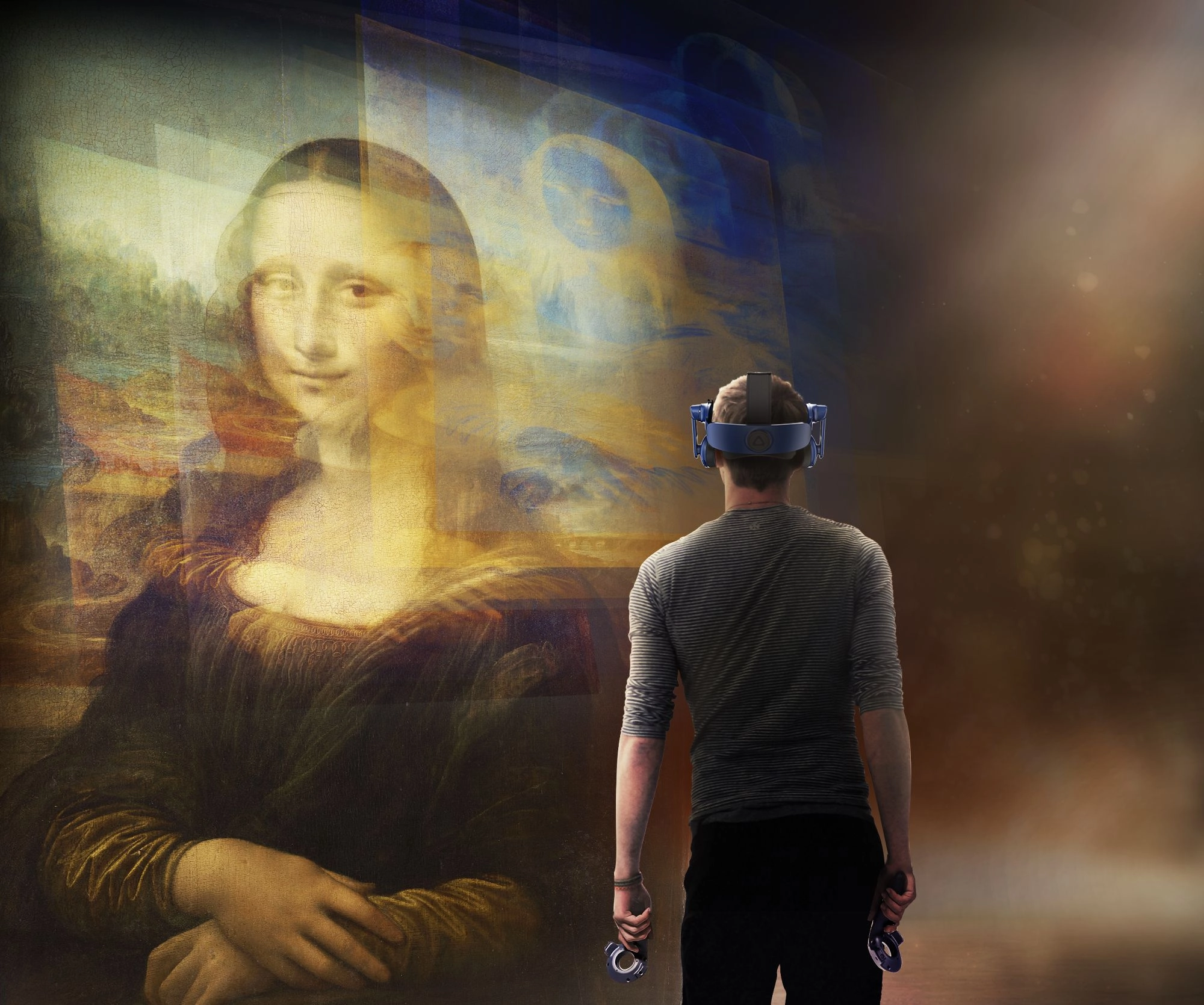The image is a heavily stylized, edited photograph that depicts a man engrossed in a virtual reality (VR) experience, centered in a rectangular frame. The man has short brown hair and wears a long-sleeve shirt with black and white horizontal stripes, its sleeves pushed up above his elbows, paired with black pants. His back faces the camera, and a large, blocky VR headset, characterized by a thick black band around the back and top of his head, is prominently worn. The headset features blue accents around the middle and sides. 

In both hands, the man holds VR controllers, which resemble handles with circular discs. The VR environment he is immersed in prominently features the Mona Lisa painting, twice his height, situated slightly to the left in the background. The image of the Mona Lisa—a woman with black hair, sitting with her hands crossed and clad in a dark robe—is somewhat blurred and overlain with other semi-transparent photos, some showing blue and yellow circles. To the right, a stream of light cuts diagonally across the scene, creating a foggy atmosphere speckled with dust particles, adding to the ethereal and immersive ambiance of the VR space.